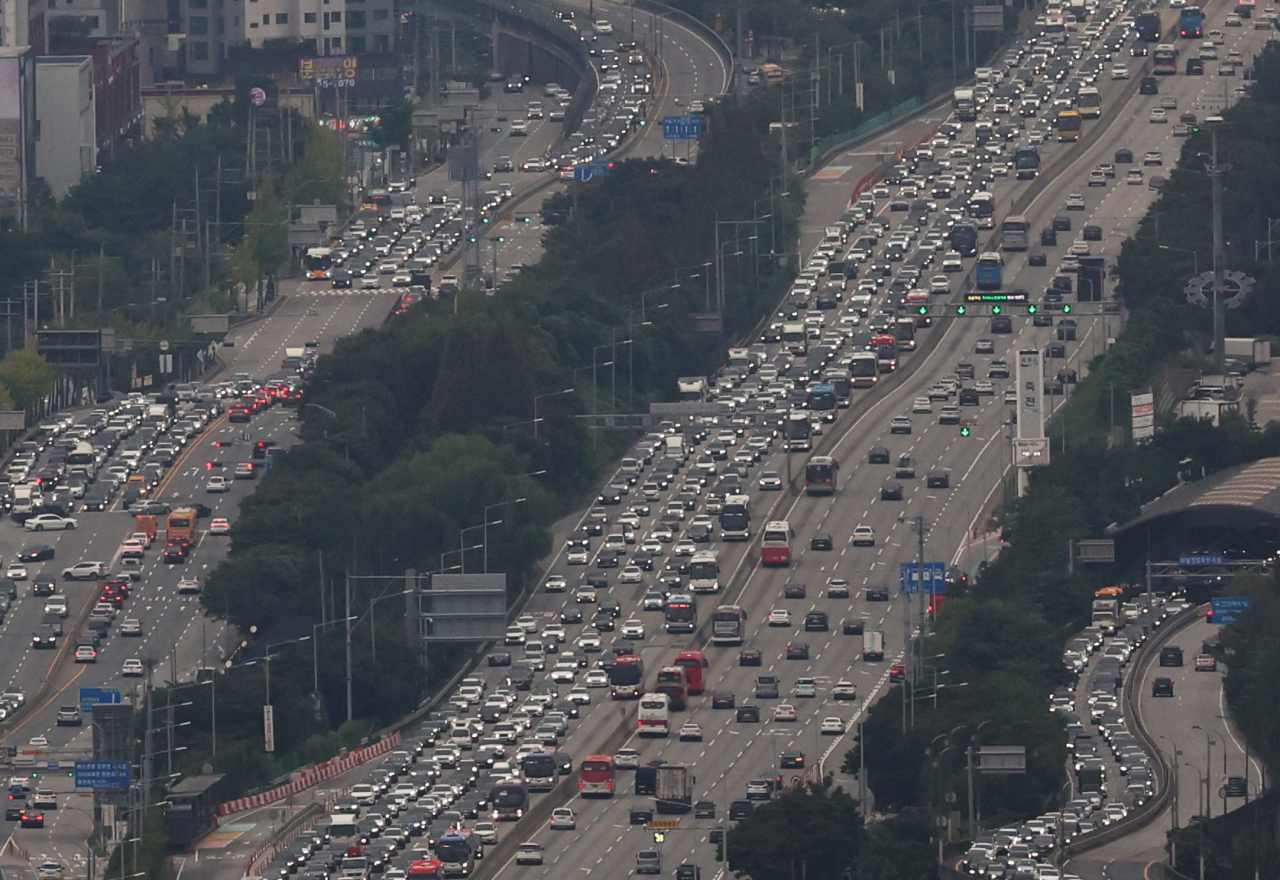This photograph, taken from an elevated perspective, captures a sprawling, highly populated city freeway system. The shot, possibly from a tower or a helicopter, looks downward towards three major parallel highways packed with vehicles. The central highway, the most prominent with ten lanes (five in each direction), stretches diagonally from the lower left to the upper right of the image. Despite the heavy traffic in both directions, the lanes towards the viewer are particularly congested, showcasing numerous cars and buses with visible brake lights. Conversely, the lanes moving away from the viewer are somewhat less crowded but still busy. Blue signs and green traffic lights are discernible along these routes, with some streetlights and power lines lining the roads. Separating these highways are strips of lush greenery, dotted with trees. On the smaller road to the right, there is a covered overpass area. Buildings are visible towards the upper left, adding to the cityscape setting of this bustling transportation network.